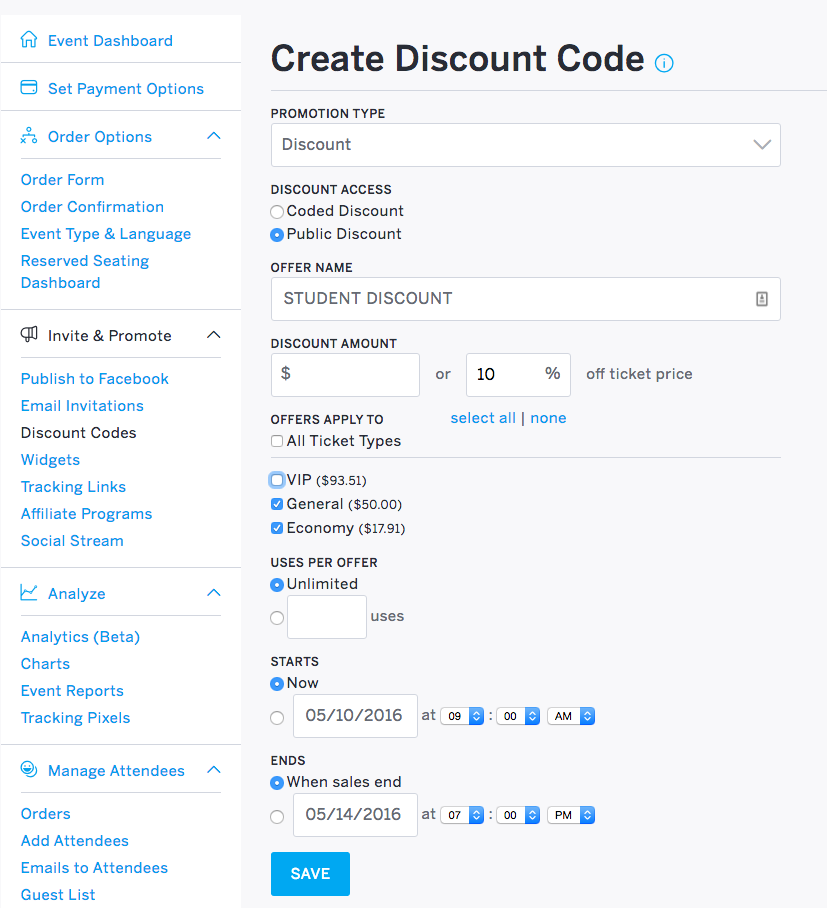In this image, we see a comprehensive dashboard designed for creating discount codes for events. The interface features a dropdown menu allowing users to specify the type of promotion—whether a coded discount or a public discount. The name of the offer is auto-filled with "Student Discount," and users can specify the discount amount either in dollar form or as a percentage off the ticket price. 

Users can apply the discount to all ticket types, including VIP, General, and Economy. Additionally, they have the option to set user limits per offer, choosing between unlimited access or a specified number of users. The dashboard also allows for precise scheduling, enabling users to define the start and end dates and times for the discount.

On the left-hand side of the dashboard, there's a well-organized column of links for various settings and options, including:

- Event Dashboard
- Payment Options
- Order Options
- Order Form
- Order Confirmation
- Event Type and Language
- Reserved Seating Dashboard
- Invite and Promote
- Publish to Facebook
- Email Invitations
- Discount Codes
- Widgets
- Tracking Links
- Affiliate Programs
- Social Stream
- Analyze section with:
  - Analytics (Beta)
  - Charts
  - Event Reports
  - Tracking Pixels
- Manage Attendees with options like:
  - Orders
  - Add Attendees
  - Email Attendees
  - Guest List

At the bottom of the interface, there's a "Save" button to preserve any modifications made. The dashboard provides an intuitive and exhaustive suite of tools for event organizers to manage discounts and various event-related settings effectively.